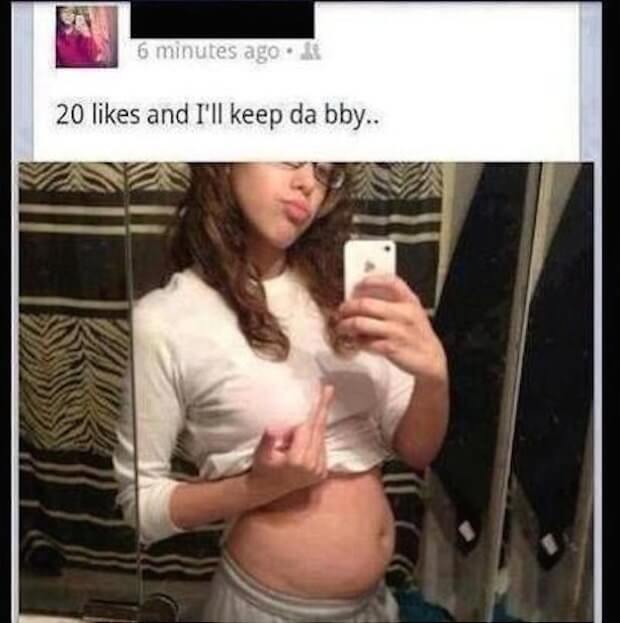The image, a social media post, portrays a young, pregnant woman taking a reflection-type selfie in a bathroom mirror. She has long brown hair, black-rimmed glasses, and wears a white long-sleeve shirt pulled up to reveal her pregnant belly, paired with light gray shorts or pants. The woman holds a white iPhone in her left hand while making an obscene gesture with her right hand. Behind her hangs a shower curtain with a black and tan pattern. Above the photo is a caption stating "20 likes and I'll keep da baby..." posted 6 minutes ago, next to the poster's profile picture, which shows a woman in a reddiresh-purple shirt. The post is designed to capture attention and provoke a reaction, asking for social validation on a deeply personal decision.